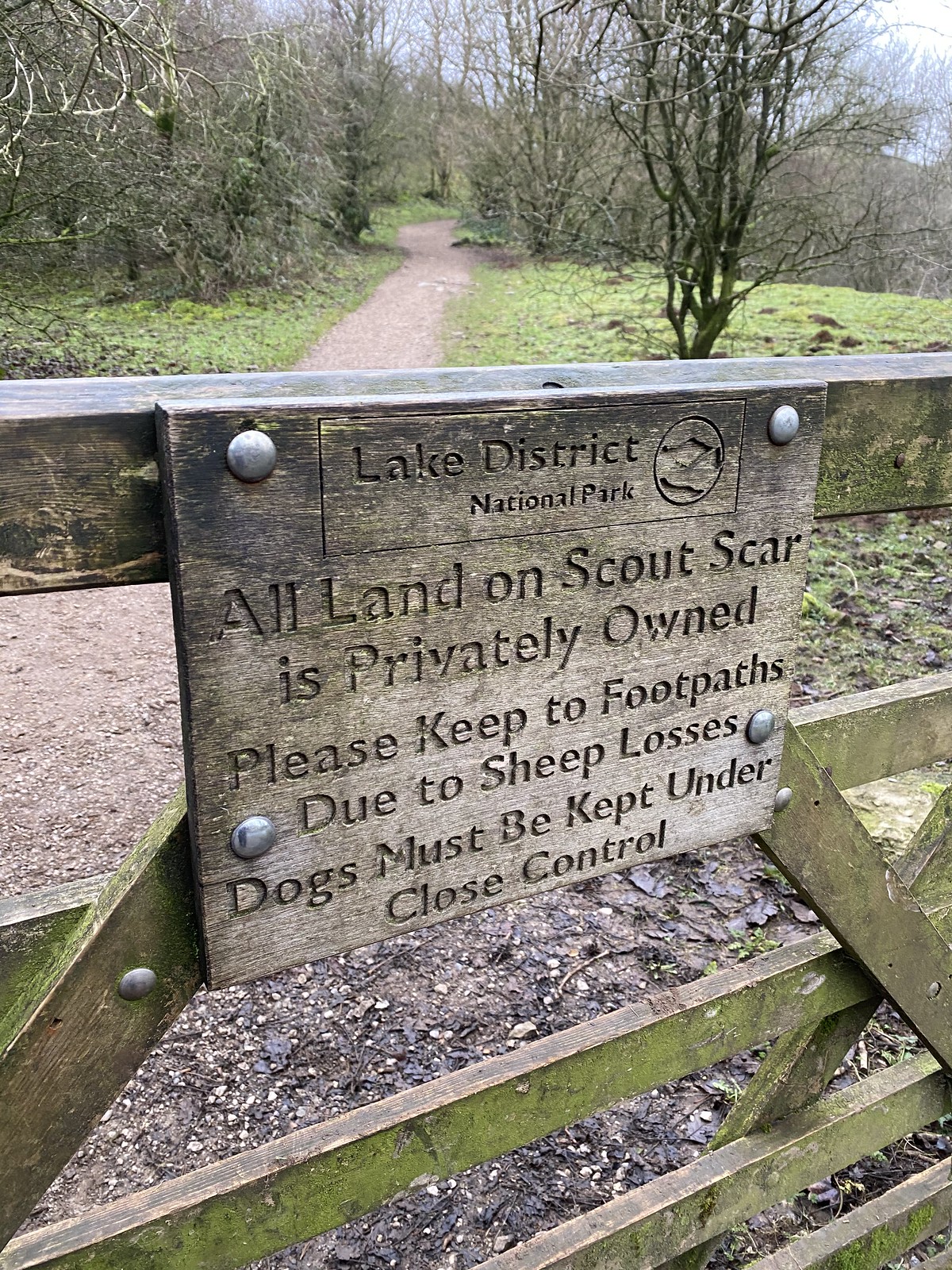The image depicts an entrance to the Lake District National Park, showcasing a rustic wooden gate bolted to a low cement wall. The gate prominently features a wooden sign etched with detailed instructions: "Lake District National Park" followed by "All land on Scout Scar is privately owned. Please keep to footpaths. Due to sheep losses, dogs must be kept under close control." The sign also includes a logo at the top. The background reveals a serene wooded area with abundant trees and a lush, green forest. A rocky and slightly uneven path meanders through the forest, providing a clear route for walkers. The sky above is blue with minimal clouds, suggesting a pleasant day. Paths are visible through the trees and bushes alongside the main track, enhancing the picturesque and inviting atmosphere of the natural landscape.